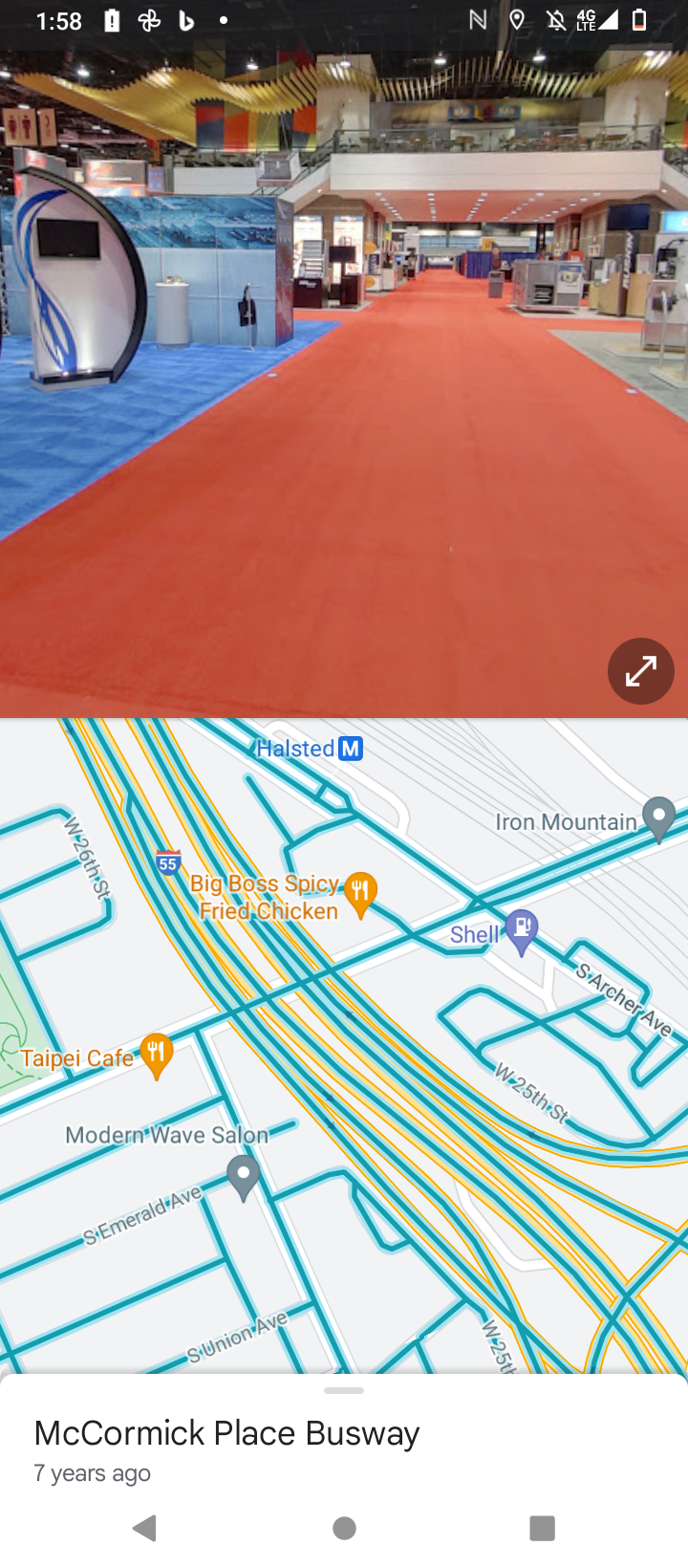The image is a vertically-oriented rectangle divided into two distinct squares. The top square is a photograph of a large public space featuring an orange carpet running down the middle, flanked by blue carpet on the left and a green carpet square on the right. Overhead, an art piece resembling a wavy bridge made of wooden slats adds an architectural intrigue to the scene. A white column with an embedded black screen or monitor is positioned on the left side. This column is surrounded by a black curved structure and a blue wavy shape, contributing to the modern aesthetic of the space.

At the top of the screenshot, the time reads 1:58, and the battery icon is nearly depleted with a red indicator, signifying low battery. The status bar also shows "4G LTE" connectivity, indicating a mobile network connection.

The bottom square of the image displays a map marked with various labeled locations, including "Modern Wave Salon," "South Emerald Ave," "Taipei Cafe," "Big Boss Spicy Fried Chicken," "Halsted," "Iron Mountain," and a "Shell" gas station. At the very bottom, the map is titled "McCormick Place Busway" in black lettering, with a note that says "7 years ago" beneath it, suggesting that the map view is from a historical perspective.